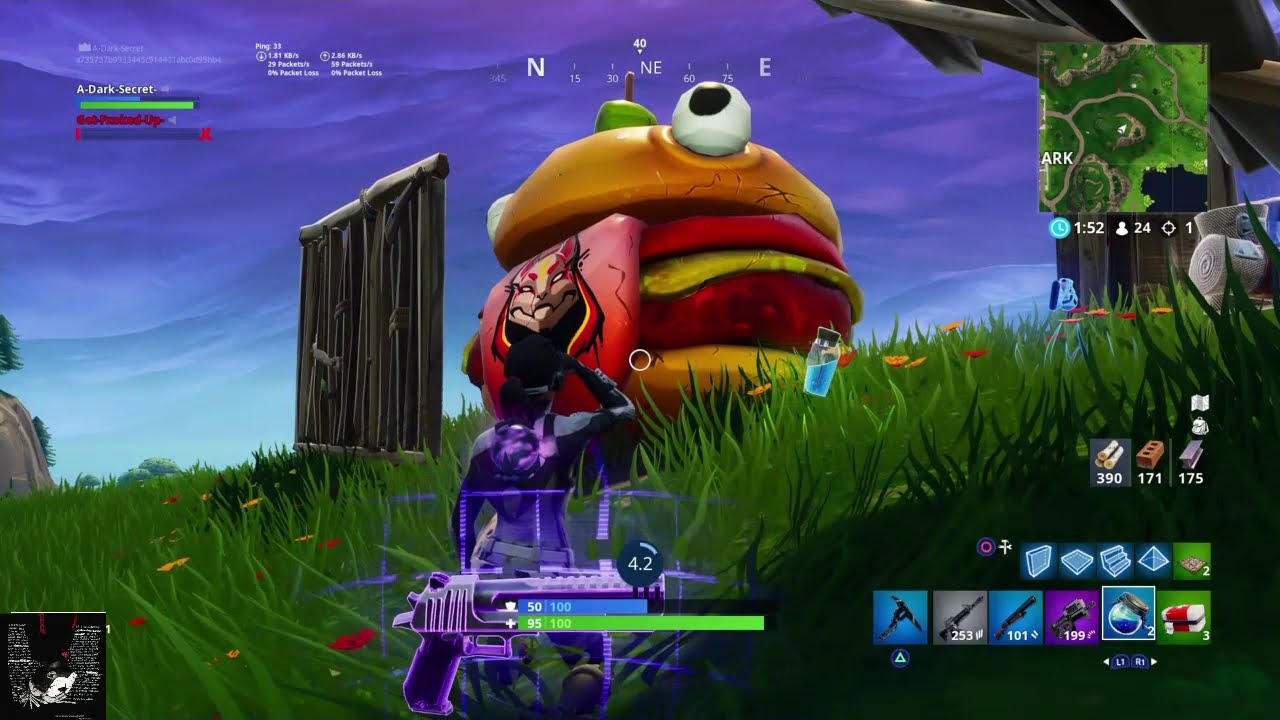The image is a screenshot from a video game, likely Fortnite, featuring vivid gameplay elements. Centered on a grassy hill, there's a giant cheeseburger creature with large, expressive eyes on its top bun and a tongue outstretched, on which rests a cat figure. In front of this peculiar burger monster stands a player character, slightly smaller, dressed in a distinctive black and purple costume, attentively looking at the cheeseburger figure. The background reveals a partially constructed fort against a blue sky dotted with clouds. The game's HUD (Heads-Up Display) is visible, with a detailed map and time in the top right corner, a compass in the top middle, and the player’s health and armor status along with available ammo and inventory options in the bottom right corner. The foreground shows the player’s current weapon choice, with a prominently displayed purple gun icon flanked by stamina bars.